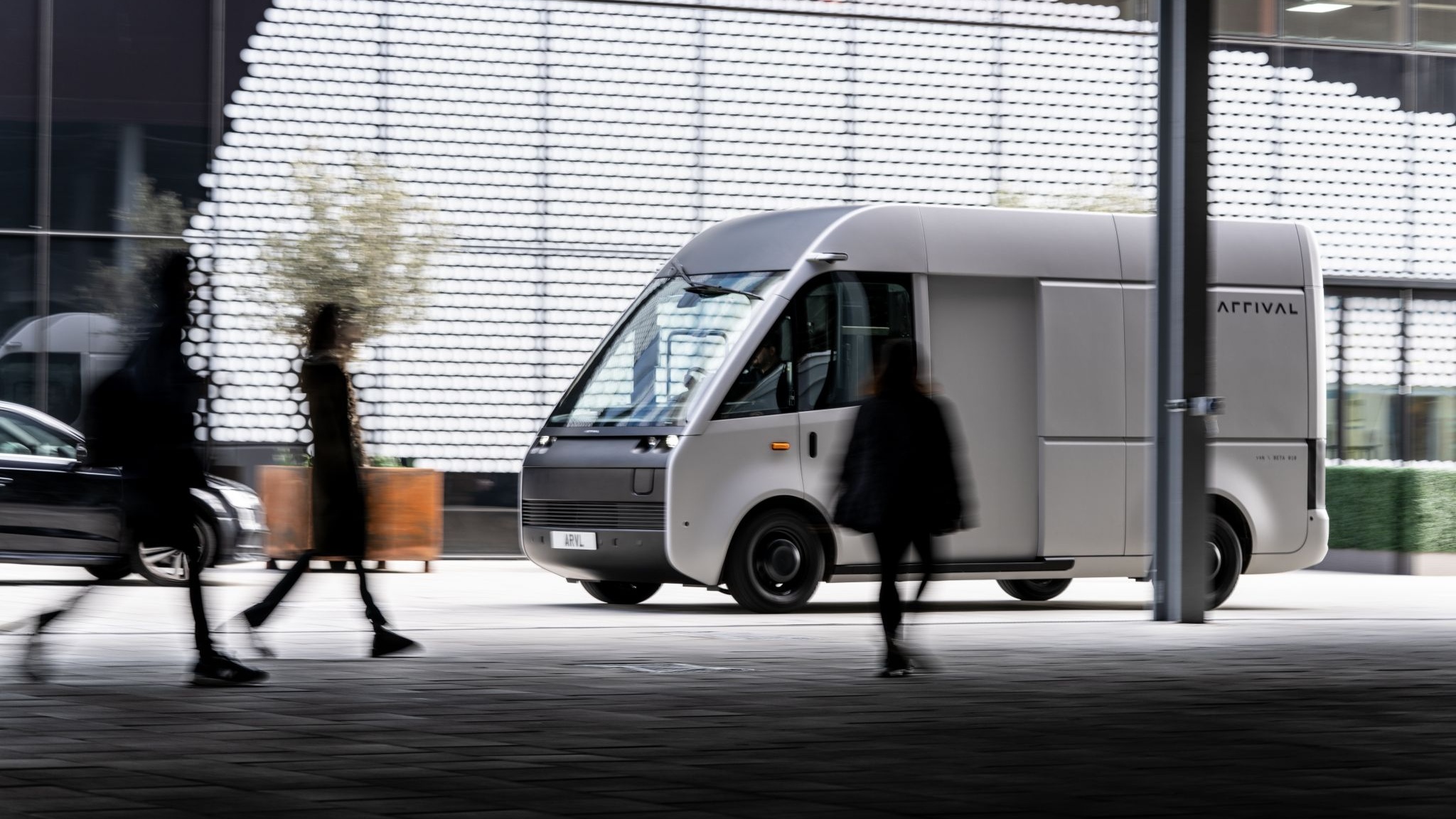This photograph/rendering showcases a futuristic grey van with black wheels, displaying the word "Arrival" in a stylish font on its rear portion. The vehicle features a sleek, angular design with a large side door and an expansive windshield that extends across the entire front, eliminating the traditional bus nose. This creates a modern, streamlined appearance. The scene is set outdoors, possibly near a busy commuter station like an airport or train station, with a perforated, metal-grated wall and a partially visible, regular car to the left. In front of the vehicle, three blurred human silhouettes are visible, contributing to the dynamic urban setting. Also blurry in the background is a green tree, highlighting the focus on the innovative electric van.